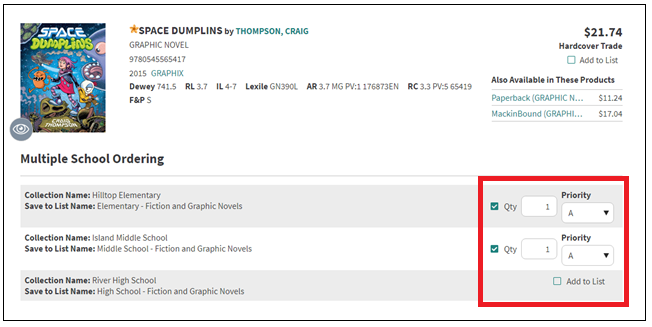This screenshot displays an online ordering interface for a book titled "Space Dumplings." The top-left corner features an image of the book, depicting a girl with striking purple-pink hair and several whimsical, cartoonish creatures that resemble an octopus. Next to the image, the book is identified as "Space Dumplings" by Thomas Craig, and it is classified as a graphic novel. The publication details note that it was released in 2015 by Graphics Dewey with the code 741.5.

To the right, further details are given:
- Hardcover price: $21.74
- Trade paperback: $11.24
- Mac and Ben graphic: $17.04

Below this information, the book appears in several school collection lists:
- Hilltop Elementary: Saved to 'Elementary Fiction and Graphic Novels'
- Island Middle School: Saved to 'Middle School Fiction and Graphic Novels'
- River High School: Saved to 'High School Fiction and Graphic Novels'

To the far right, a red square labeled "Priority" indicates that a single copy of the book has been checked for order.